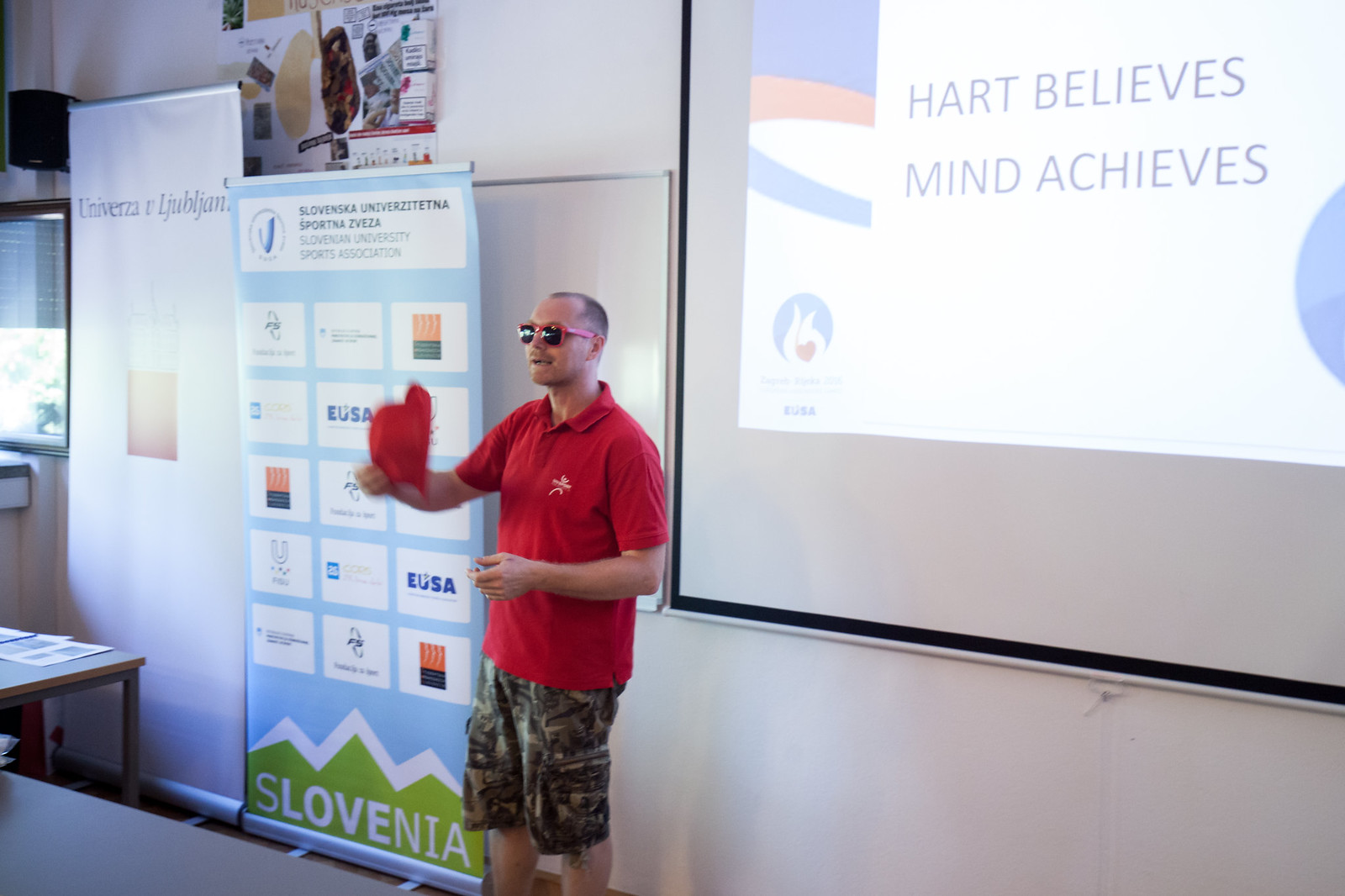A man stands in front of a digital display, facing to the left with his hands held out in front of him, holding a red cap in one hand. He is dressed in a red short-sleeved polo shirt with a white emblem on the chest and wears pink sunglasses and camouflaged shorts that extend below his knees. He has short black hair and a slight smile on his face. The background features a white wall, suggesting a classroom setting. Behind him, to the right, the digital display has a white box with the words "Heart Believes, Mind Achieves" surrounded by a black trim. To the left of the man, another banner with a light blue background and several white squares and rectangles is visible. The bottom section of the banner has a green background with sharp mountain shapes and white text that reads "Slovenia," indicating a possible educational setting in a Slovenian institution.